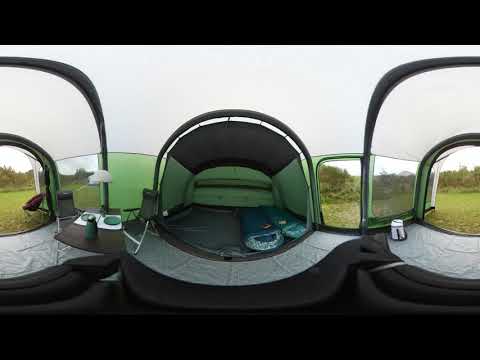This image captures the panoramic interior and surroundings of a green and gray tent from a 360-degree perspective. Central to the photograph is the tent's entrance, which showcases the tent's inviting opening, allowing a glimpse outside to a grassy area with a sprinkling of bushes and distant trees. The interior features a green fabric wall that curves up to meet a mesh material ceiling, providing ventilation and a soft influx of light. Inside, right in the middle of the tent floor, lies a green sleeping bag, evoking the snug feel of a large, comfy pencil case. Adjacent to this is another sleeping bag, blue in color, emphasizing the tent's preparation for multiple campers.

To the sides of the sleeping bags, several camping essentials are neatly arranged. A small floating chair with a green canvas seat and metal frame sits off towards one side, suggesting a spot for relaxation or reading. Nearby, a white box carrier with handles, potentially used for storage, is visible, adding to the campsite organization. All the way to the left, a little table area is noticed, potentially holding a plate and a container, indicating a space for meal preparations or quick snacks.

Overall, this detailed panorama encapsulates the cozy, well-equipped interior of a tent set against the backdrop of a pleasant day with green grass and distant trees, painting a serene and organized camping scene.